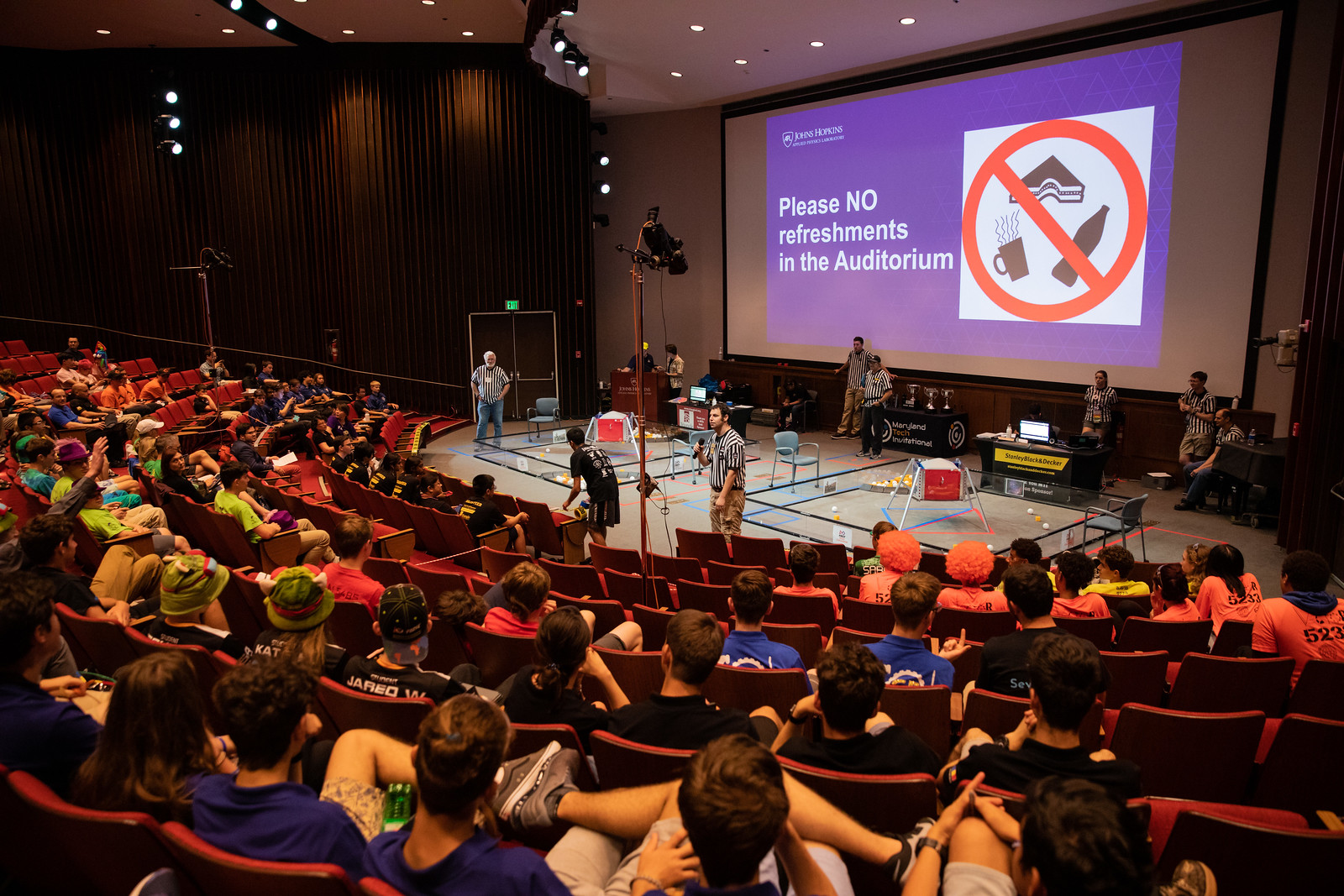This image captures a lively lecture or assembly, likely a college-level competition, set in an auditorium featuring stadium seating with red chairs. The audience, mainly composed of teenagers or young adults, suggests a university-like environment, possibly Maryland Tech or Johns Hopkins, as indicated by the differing mentions of the institutions. The stage, positioned in front of a light tan backdrop, is bustling with activity. 

A prominent large projection screen dominates the background, displaying a blue or purple notice that reads, "Please No Refreshments in the Auditorium," accompanied by icons of forbidden items like a sandwich, a cup of coffee, and a bottle, each crossed out with a red circle and slash.

On the stage, several referees dressed in black and white striped uniforms oversee the event, hinting at a structured competition. The stage features two side-by-side contraptions enclosed in short plexiglass barriers, each containing a suspended red and white basket supported by a metal frame, suggesting a science-related challenge or game.

At the forefront, on the right side of the auditorium, a group of participants clad in matching pink T-shirts and pink wigs sit together, likely one of the competing teams. In addition, a table draped with a banner reading "Maryland Tech Invitational" is adorned with three large trophies, reinforcing the competitive nature of the gathering.

The overall ambiance is one of excitement and anticipation, with an auditorium about 75% full, indicating a well-attended event in which hundreds of spectators engage with enthusiasm and compliance with basic rules, as reiterated by the projection screen's reminder.